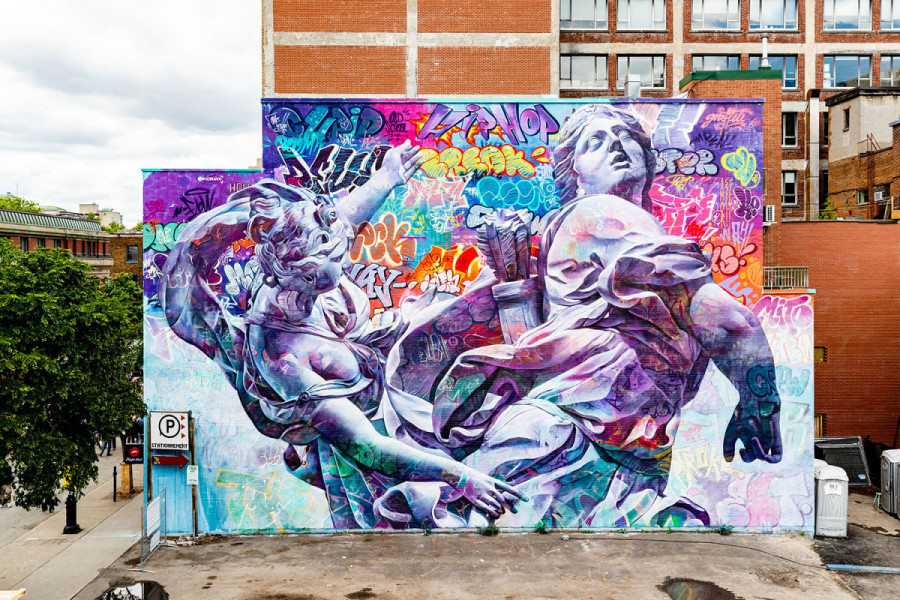In this outdoor scene, a captivating mural stretches across the side of an orange brick building with a gray roof and large windows. The mural, a blend of classical and modern elements, overlays vibrant graffiti featuring names and words in colorful, curvy letters. The central focus is two Greek or Victorian-style figures rendered in striking white and purple hues. The prominent figure on the right is a muscular, Victorian-era woman clad in a loosely draped t-shirt and equipped with a quiver of arrows slung across her back. Facing her is a shorter figure, also in a classical style, partially obscured and seemingly reaching out to touch the taller woman's right leg. The scene is set against a backdrop of trees and a cloudy sky, with another orange building to the left and a red building visible at the top right. The mural's intricate details and the fusion of historical imagery with modern graffiti create a dynamic and visually engaging work of art.